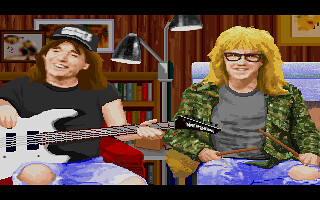In this 8-bit vintage-style still from the Wayne's World video game for Super Nintendo, the scene is set in Wayne's basement, depicted with wood-paneled walls, a bookcase, and small pictures. Wayne, situated on the left, sports a black t-shirt and ripped blue jeans, along with a black hat emblazoned with "Wayne's World." He holds a white guitar, gripping the top with his left hand and supporting the bottom with his right, while seated on a red couch. 

Adjacent to Wayne, a double light lamp stands with two bulbs – one extending to the left and the other to the right, with the right bulb slightly taller. To the right is Garth, characterized by his black-rimmed glasses, military camouflage jacket over a gray t-shirt, and blue jeans with a tear on the left knee. He sits while clutching drumsticks. This detailed portrayal of the iconic duo captures the nostalgic ambiance of their basement hangout.